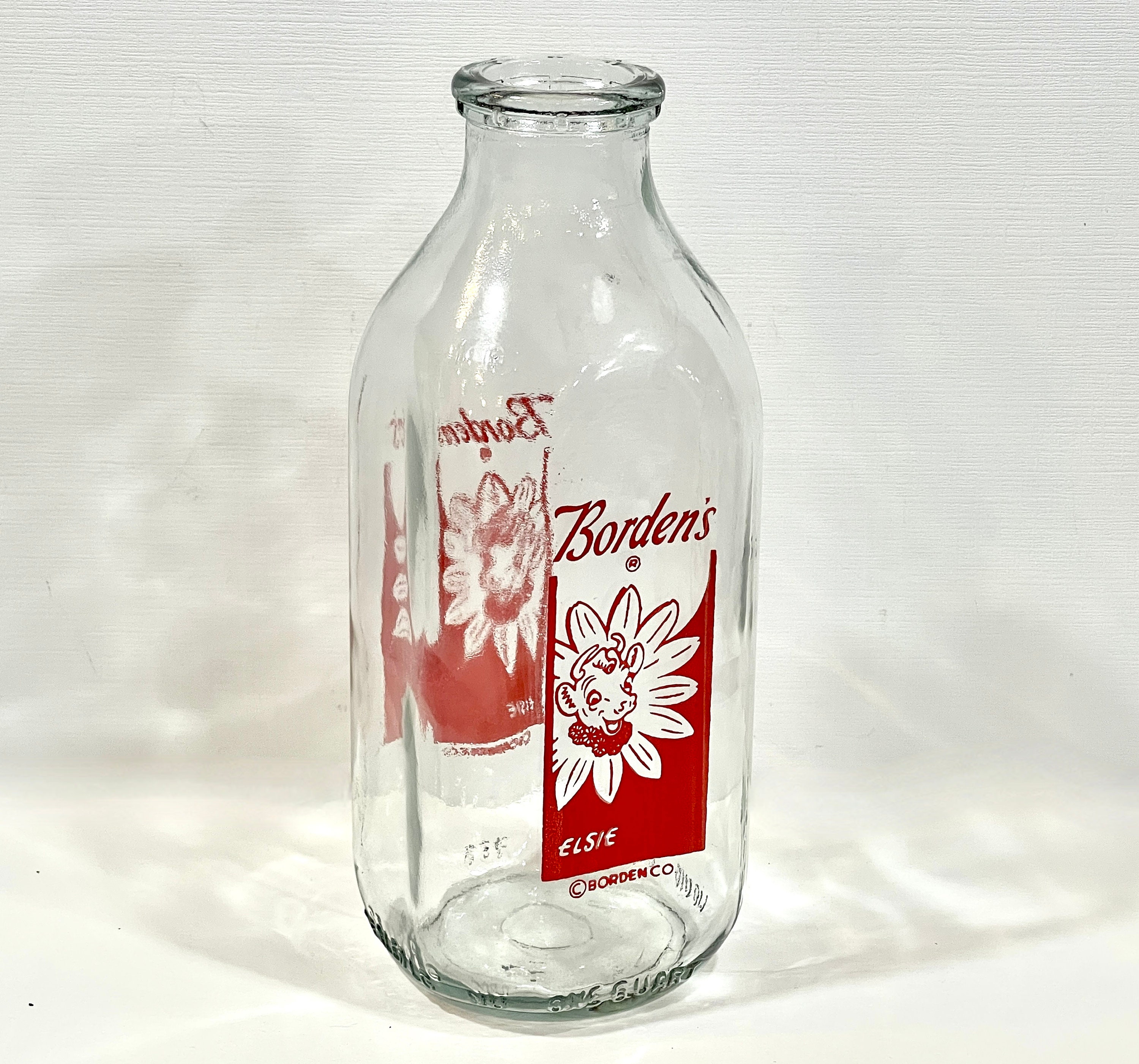This photograph showcases a vintage glass milk bottle, likely from the 1930s or 1940s, set against a flat white surface and a white background. The cylindrical bottle narrows into a short neck with a slight outward glass rim at the top and lacks a lid. Prominently featured is the iconic Borden's dairy logo on both the front and the back, which can be faintly seen through the glass. The logo is displayed within a vertical rectangle and consists of the word "Borden's" in italic red print at the top, followed by a small red circled "R". Below is a white circle encasing the head of a smiling cow, adorned with a daisy wreath. The cow, outlined in red, has its mouth open and sports horns along with a curly tuft of hair. Directly beneath the cow, set against a red background, is the name "Elsie" in handwritten white text, referring to the beloved Borden dairy mascot. Toward the bottom of the logo is the text "C Borden CO." This meticulous detail encapsulates the charm and history of this nostalgic dairy artifact.